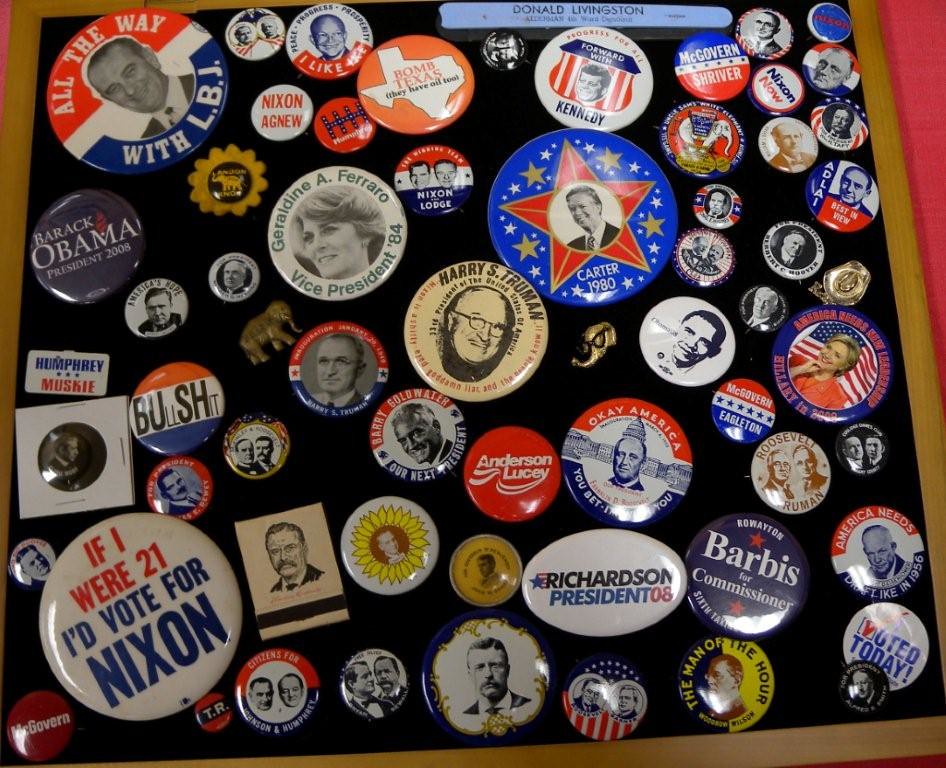This image showcases a detailed display case filled with a vast collection of presidential campaign buttons, prominently framed in light wood against a black background. The buttons span various U.S. presidential campaigns, featuring notable figures such as Richard Nixon, John F. Kennedy, Barack Obama, Lyndon B. Johnson (LBJ), Harry S. Truman, and Theodore Roosevelt, among others. Noteworthy buttons include "If I were 21, I'd vote for Nixon," "All the way with LBJ," and a humorous one spelling "B-U-L-L-S-H-I-T" for Bush. The collection, estimated to contain around 20-30 buttons, varies in size and design, with some adorned with American flags and state-themed motifs. Additionally, there are pins, including one depicting elephants, and other election memorabilia like matches. The overall presentation is meticulous, making it clear that this assemblage is a treasured showcase of political history.